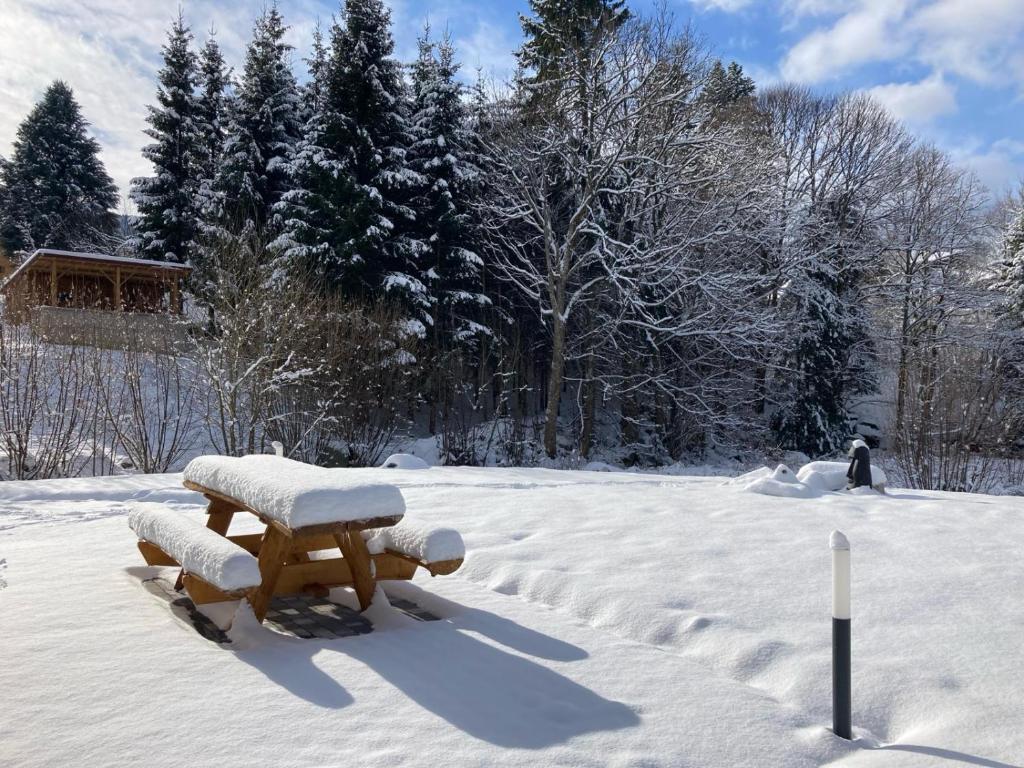This image captures a serene outdoor winter scene in the countryside, centered around a small wooden cabin nestled on a slight hill towards the left. The cabin, with its faint blanket of snow on the roof, is surrounded by a mix of tall evergreen trees and barren trees, all draped in thick, fluffy snow. The evergreens stand proudly against a backdrop of a vibrant blue sky filled with large, white clouds. At the forefront, the ground is covered in a pure, untouched layer of deep, soft snow, highlighting the idyllic and undisturbed nature of the setting.

A picnic table, positioned prominently in the foreground, is laden with about a foot of snow, its wooden parts still visible beneath the weight. Beneath the blanket of snow, a walkway subtly divides the scene, leading to a small gray and white post at its end. Close by, there appears to be another indistinct snowy object, possibly a statue, standing quietly towards the edge of the forested area. The scene evokes a sense of tranquility and natural beauty, emphasizing the peaceful isolation of this snow-covered landscape.